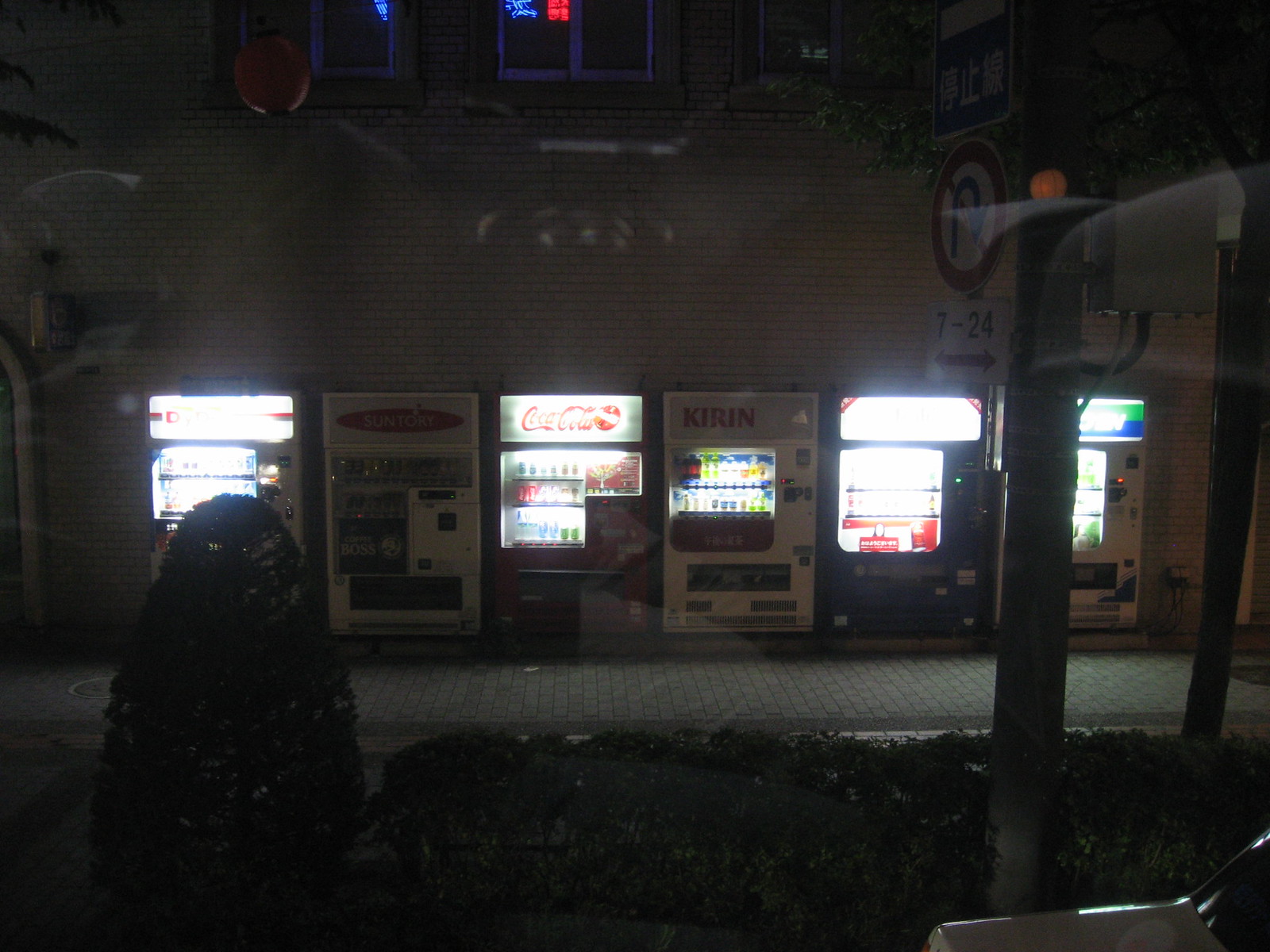This nighttime photograph, likely taken through a window, captures a row of six vending machines situated across a dimly-lit street. The reflections on the glass add an extra layer of depth to the vibrant scene. The vending machines are of substantial size and width, with various brandings and logo displays. Starting from the left:

1. The first and fourth vending machines have their screens glowing so intensely that the displayed content is indistinguishable, presenting as bright blurs.
2. The second machine stands out with a clear Suntory logo set in a red oval.
3. The third machine prominently features the Coca-Cola brand, with visible glass bottles of Coca-Cola products.
4. The fifth machine is branded with Kirin, showcasing its selections against a backdrop that resembles a blue sky.
5. The sixth machine has a white exterior with a green and blue sign, its selections also illuminated.

Further in the background, there is a building with a wooden board and signage indicating traffic regulations, such as a "no U-turn" sign for 7-24 hours. A small bush is visible at the bottom left, adding a touch of greenery to the urban scene.